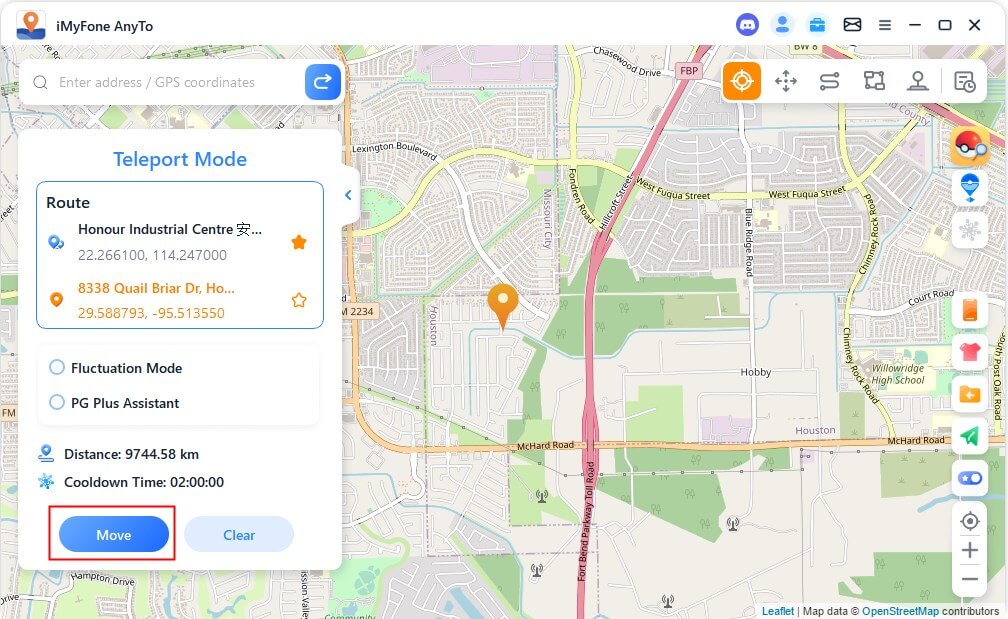### Detailed Screenshot Description

The image is a screenshot of a mobile application interface, likely related to location tracking or GPS functionality. Here's a detailed breakdown of the different elements present on the screen:

#### Top of the Screen
- **Icon in the Upper Left Corner**: An orange pin marker icon over a blue terrain with a white sky.
- **App Name**: Displays "MyFone AnyTo".
- **Icons on the Upper Right Corner**:
  - **Discord Logo**: A purple disc with a white graphic in the center.
  - **Middle Icon**: Unidentified white detail in the center.
  - **Profile Icon**: Dark blue icon on a light blue background.
  - **Briefcase Icon**: Dark blue icon on a light blue background.
  - **Additional Icons**: 
    - Black icons on a white background representing an envelope, three-bar menu, single bar, square, and an X.

#### Map Area
- **Background**: A map displaying an area where Missouri City and Houston intersect.

#### Left Side
- **Search Bar**:
  - White bar with gray text and a magnifying glass icon.
  - Text reads "Enter address/GPS coordinates".
  - A blue button with a white U-turn arrow labeled "Go".

#### Main Information Box
- **Title**: "Teleport Mode" displayed in blue text.
- **Route Box**: Lists two waypoints.
  - **First Waypoint**:
    - Label: "Honor Industrial Center" followed by Chinese characters.
    - Coordinates: 22.266100, 114.247000.
    - Map Markers: Two blue markers (one smaller in the background, one larger in the foreground) on the left.
    - Orange star filled in on the right.
  - **Second Waypoint**:
    - Label: "8338 Quail Briar Drive, HO..." (cut-off text).
    - Coordinates: 29.588793, -95.513550.
    - Single map marker in orange.
    - Orange star not filled in on the right.

#### Options and Indicators
- **Selection Options**: Within a light gray-bordered box.
  - **Radio Buttons**:
    - "Fluctuation Mode"
    - "PG+ Assistance"
- **Additional Route Information**:
  - Black map marker with a line beneath (route indicator).
  - Text: "Distance: 9744.58 kilometers".
  - Small snowflake icon with blue text indicating "Cool Down Time: 020000" (interpreted here as potentially 2 hours).

#### Buttons at the Bottom
- **Red Box Surrounding Blue Button**: White text "Move".
- **Light Blue Button**: Dark blue text "Clear".

This thoroughly captures the intricate details and functionality presented within the screenshot.